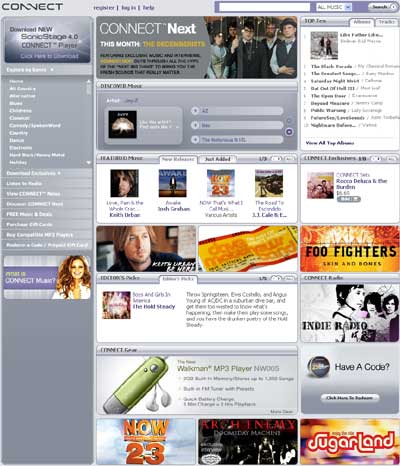The image depicts an old music website named "Connect," characterized by its highly pixelated and blurry interface. At the top of the site, there are options for users to "Register" and "Log In." The central feature showcased is a prompt to "Download Sonic Stage 4.5 Connect Player," hinting that this platform was used extensively in the past for acquiring music. The website's main navigation includes sections such as "Discovery Music," with an area to input user information.

On the right-hand side, there's a top 10 list of songs, although the exact titles are obscured due to the blurriness. Featured prominently is a section labeled "Highlighted Music," which is currently displaying the "New Releases" tab. This section includes various music albums along with their covers, mentioning artists like the Foo Fighters with their album "Skin and Bones," and another artist, possibly Keri Murray, whose name is also hard to decipher.

Additionally, the sidebar includes an image of a ticket stub and a prompt for “Indie Radio” where visitors can “Have a code? Click here to purchase.” There is also a promotion for a “Walkman MP3 player” on display. The bottom section of the site is populated with several album covers, further emphasizing the music-centric focus of the platform.